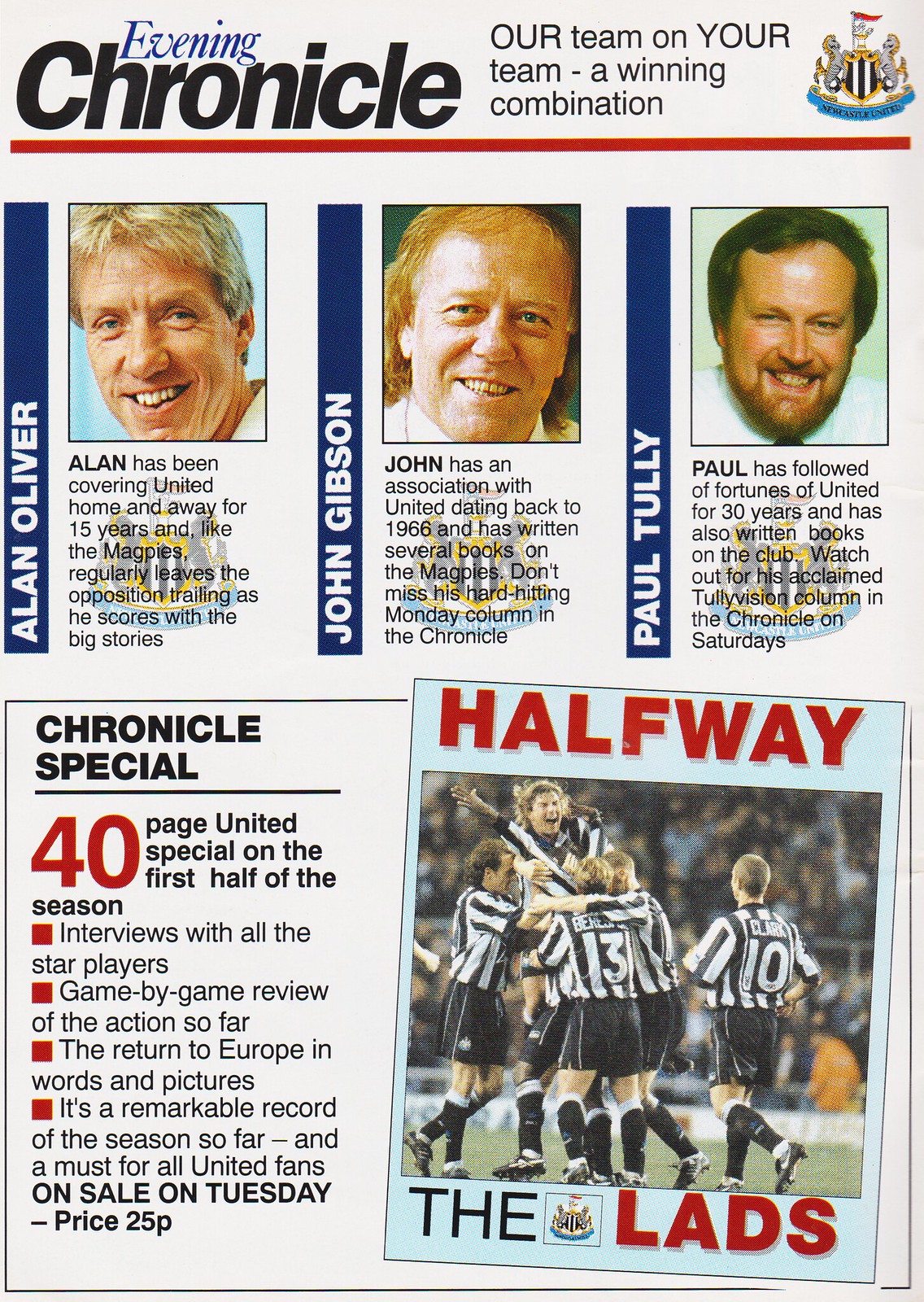The image is a page from a sports magazine with a white, aged background, headlined by the text "Evening Chronicle" in blue and black. To the right of the title, in black, it reads, "Our Team On Your Team, A Winning Combination," accompanied by a small shield-like logo in the upper right corner. Below the title, the page features three photos of men: Alan Oliver, John Gibson, and Paul Tully. Each man's photo is accompanied by a snippet of text highlighting their association with United. Alan Oliver has been covering United, both home and away, for 15 years and consistently delivers big stories. John Gibson has been connected with United since 1966, has authored several books on the Magpies, and writes a hard-hitting column every Monday in the Chronicle. Paul Tully has been chronicling United's fortunes for 30 years, has also written books on the club, and his acclaimed column, Tully Vision, appears in the Chronicle on Saturdays. Below these profiles, a photo of players in black and white uniforms lifting a teammate is prominently displayed. To the left of this image, text in black announces the "Chronicle Special," a 40-page United special on the first half of the season, including star player profiles, game-by-game action reviews, and a collection of pictures documenting the season so far. This special edition, described as a must-have for all United fans, is available on Tuesday for $25.